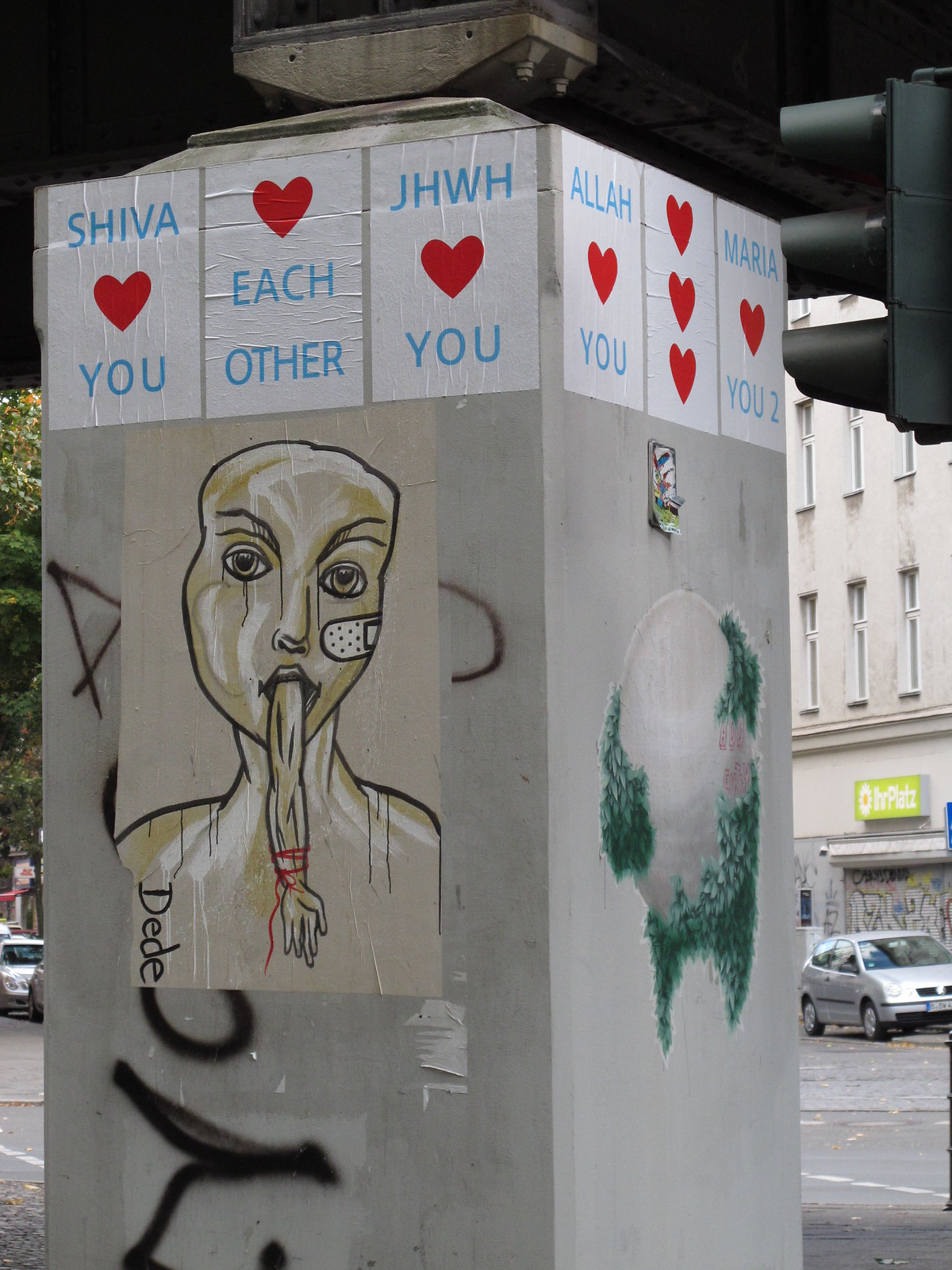In this detailed outdoor photograph, the focal point is a central concrete support pillar that holds up a bridge or overpass. The pillar is rectangular and is viewed from an angle, revealing two of its sides. Affixed to the top of the pillar are several white printer papers featuring solid red hearts and blue text. The visible messages include: "Shiva ❤ you," "❤ each other," "J H W H ❤ you," "Allah ❤ you," and "Maria ❤ you too." These heartfelt messages wrap around the visible sides of the pillar.

Below these notes, on the left side, is a piece of graffiti art depicting a primitive-looking figure with no ears, a band-aid across one cheek, and an arm emerging from its mouth. The artist's tag, "D D D E D E," is inscribed at the base of this artwork. To the right, there is another graffiti detail: a swirling white globe-like shape adorned with what appears to be patches of moss hanging down.

The setting includes an asphalt road with parked cars beside it, a building with additional graffiti, and some trees. A traffic light is visible in the upper right corner of the image, enhancing the urban atmosphere beneath the overpass. The color palette of the scene includes black, white, light blue, red, tan, gray, and green, lending it a diverse yet cohesive look.